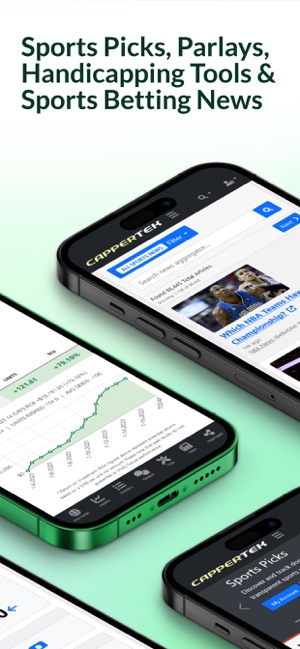This advertisement features a vertically oriented graphic with a gradient background that transitions from white at the top to green at the bottom. The prominent black text at the top reads, "Sports Picks, Parlays, Handicapping Tools, and Sports Betting News." Below the text, the design showcases four smartphones arranged in a fragmented pattern, each partially visible and displaying elements related to sports betting. Two of the phones prominently feature the logo "Capper Tech." One phone, identifiable by its green edge, displays a green-themed chart, while the other phones have black edges and show various sports betting interfaces, including an NBA team image and textual content related to sports picks. The overall composition suggests a modern, visually appealing advertisement likely intended for promoting a sports betting app, blending realistic photographs of phones with graphic design elements.